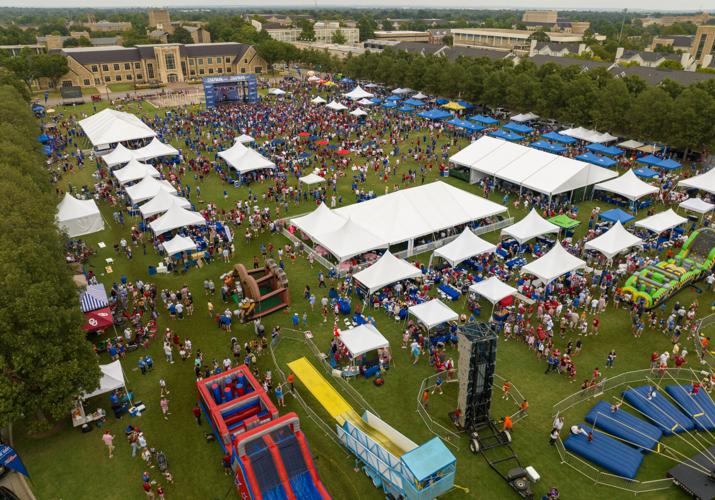This horizontally aligned rectangular aerial view captures a bustling outdoor festival, possibly at a college university. The scene is set on a large, green field flanked by rows of trees. The field is dotted with a multitude of tents: numerous smaller white tents interspersed with blue and yellow ones, and a couple of larger white tents. A crowd of people, many wearing red, white, and blue shirts, navigates through the tents and various attractions.

In the lower right corner, several blue rafts can be seen lying on the grass, hinting at possible water games or activities. On the lower left side, there is a prominent yellow slide alongside a bounce house equipped with two slides and various obstacles, indicating entertainment tailored for children. Additional inflatable rides and carnival-style games are spread across the field.

The background reveals a series of two-story, light brown stone buildings with windows, characteristic of a college campus. A particularly large gray stone building with a brown tile roof is located at the top left of the image. Toward the top left, adjacent to this building, a blue stage is set up, implying live performances or presentations might be part of the event. A sliver of cloudy sky is visible just above the buildings, suggesting overcast weather. Overall, the photograph captures a vibrant and busy event filled with activities and people.